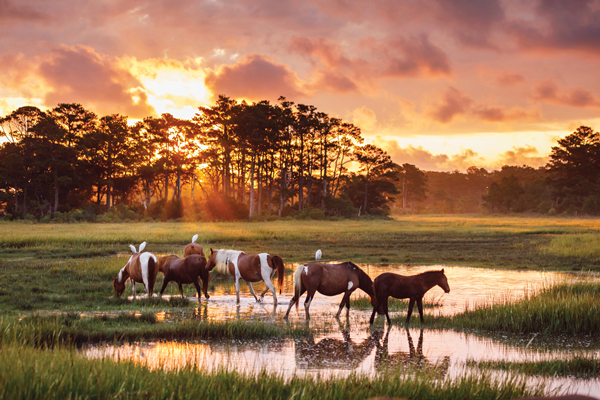In this detailed rectangular outdoor photograph, six horses are pictured in a swampy field during sunset. The swampy area features standing water that reflects the sky above and creates mirror images of the horses and dense surrounding grasses. The water level is just above the horses' hooves, and various shades of dark rain clouds fill the sky, contrasting with rays of the evening sun that peek through a row of tall trees on the top left of the image. This sunlight casts an orange-white glow over the scene, illuminating the horses and adding glimmers to the standing water below.

The horses vary in appearance; three are solid dark brown and three are painted horses with brown and white sections. One painted horse has a distinctive white tail paired with a dark mane, while another sports a dark tail and white mane. A few of the horses are leaning down to drink from the water, while others seem to be munching on grass that grows in the swampy patch. Adding to the natural harmony of the scene, four white birds are perched on the horses, blending seamlessly with the intricate setting. The serene and still beauty of the landscape, combined with the reflective water and grazing horses, offers a captivating glimpse into the wild.